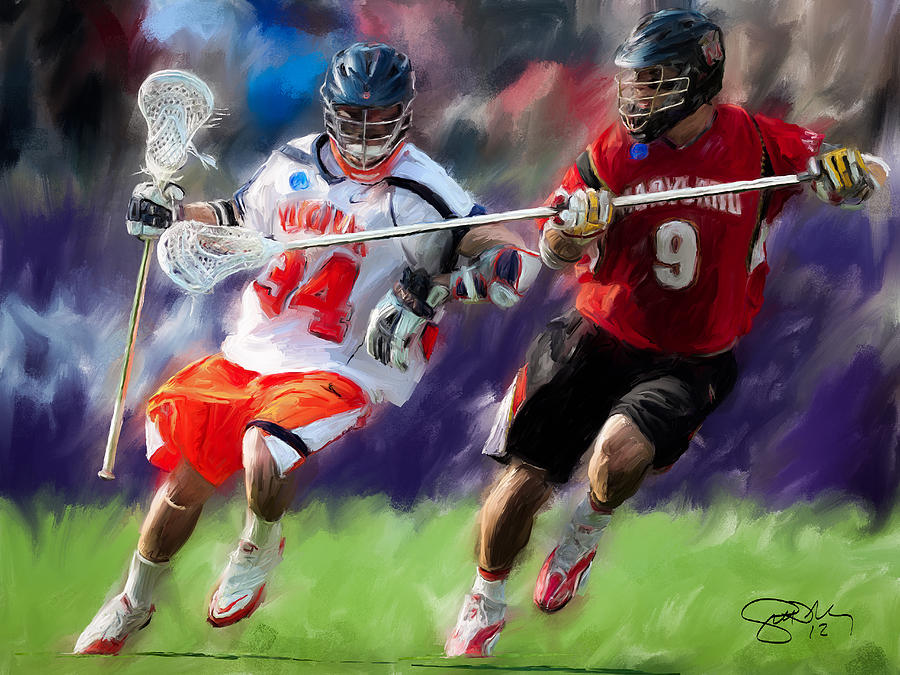This detailed watercolor painting captures the dynamic motion of two lacrosse players on the field. The background is an artistic blur of purple, gray, and blue brushstrokes, focusing attention on the central figures. The player on the right wears a red jersey with the number 9, paired with black shorts and white shoes accented with red. He sports white and yellow gloves, a black helmet, and wields a lacrosse stick with a net. The player on the left dons a white jersey with the number 34, orange shorts, and white and red tennis shoes. His gear includes white and black gloves, a black helmet, and a lacrosse stick. Notably, the painting is signed by the artist in cursive at the bottom right corner, alongside the number 12, indicating it was likely created in 2012.